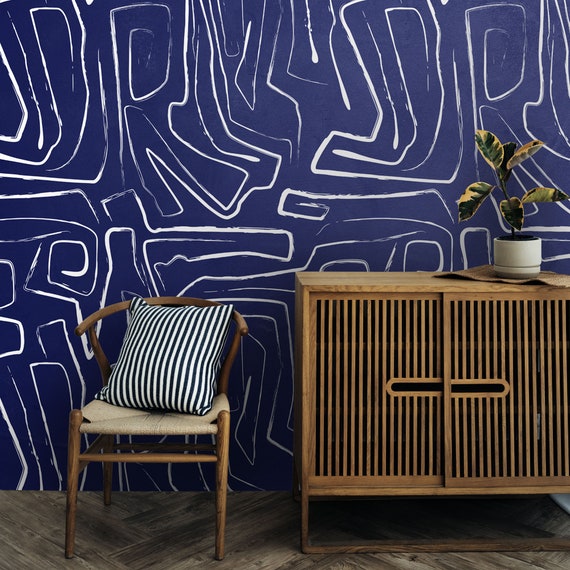In this detailed, up-close view of a modernized vanity set, the scene features a wooden chair and a small dresser against a navy blue wall adorned with abstract white calligraphy-like patterns. The chair has an open back frame made of old mahogany wood and is cushioned by a distinctive black and white zebra-striped pillow. The cozy seat of the chair is beige, and the back support appears to be made of a mesh-like material. Adjacent to the chair, the small dresser, or vanity set, constructed of light brown wood, features vertical black stripes that alternate with wooden slats. The doors of the dresser can be opened through a handhold slot. Atop this dresser sits a small ivory-colored pot housing a plant with thick leaves in vibrant shades of green and yellow. The flooring is a criss-cross pattern of wood vinyl, adding to the modern yet warm ambiance of the space.